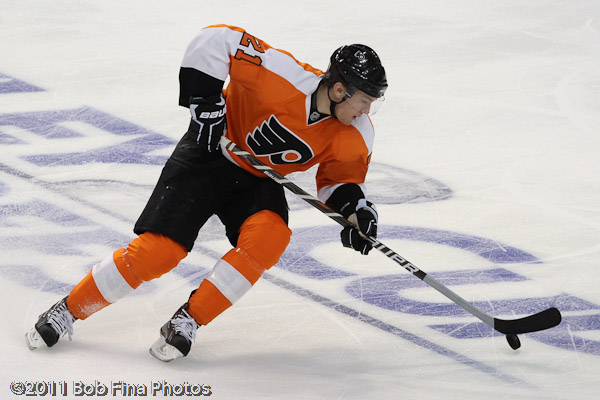The image depicts a Philadelphia Flyers hockey player, identified by the team logo on the center of his orange jersey, which features large white stripes along the shoulders and arms. He wears a black helmet, black shorts over orange pants with white stripes, and black pants. The player, number 21, is captured in action, leaning forward as he skates on the ice while dribbling a black hockey puck with his gray and black hockey stick. The ice surface, dotted with gouges and scrapes, serves as the background, featuring blue text that likely reads "Stanley Cup," although partially obscured with visible letters 'EY' and 'CUP'. In the bottom left corner of the image, a copyright notice reads "2011 Bob Fina Photos."